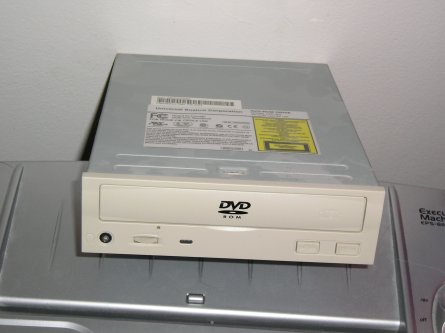This detailed photograph showcases a horizontally positioned DVD player, colored in a light off-white or silver hue, prominently sitting atop another silver electronic device, which could be a laptop or a specialized machine labeled "XMATCH." The DVD player, notable for its larger-than-typical size, is centrally featured against a white or gray wall backdrop. On the front panel of the DVD player, the text "DVD" and "ROM" is clearly visible in black letters. There are also dials and buttons located on the lower right side of the front face. The top of the DVD player is adorned with a yellow label displaying a QR code, alongside a white label containing technical specifications and additional black text, although the fine print is difficult to discern.